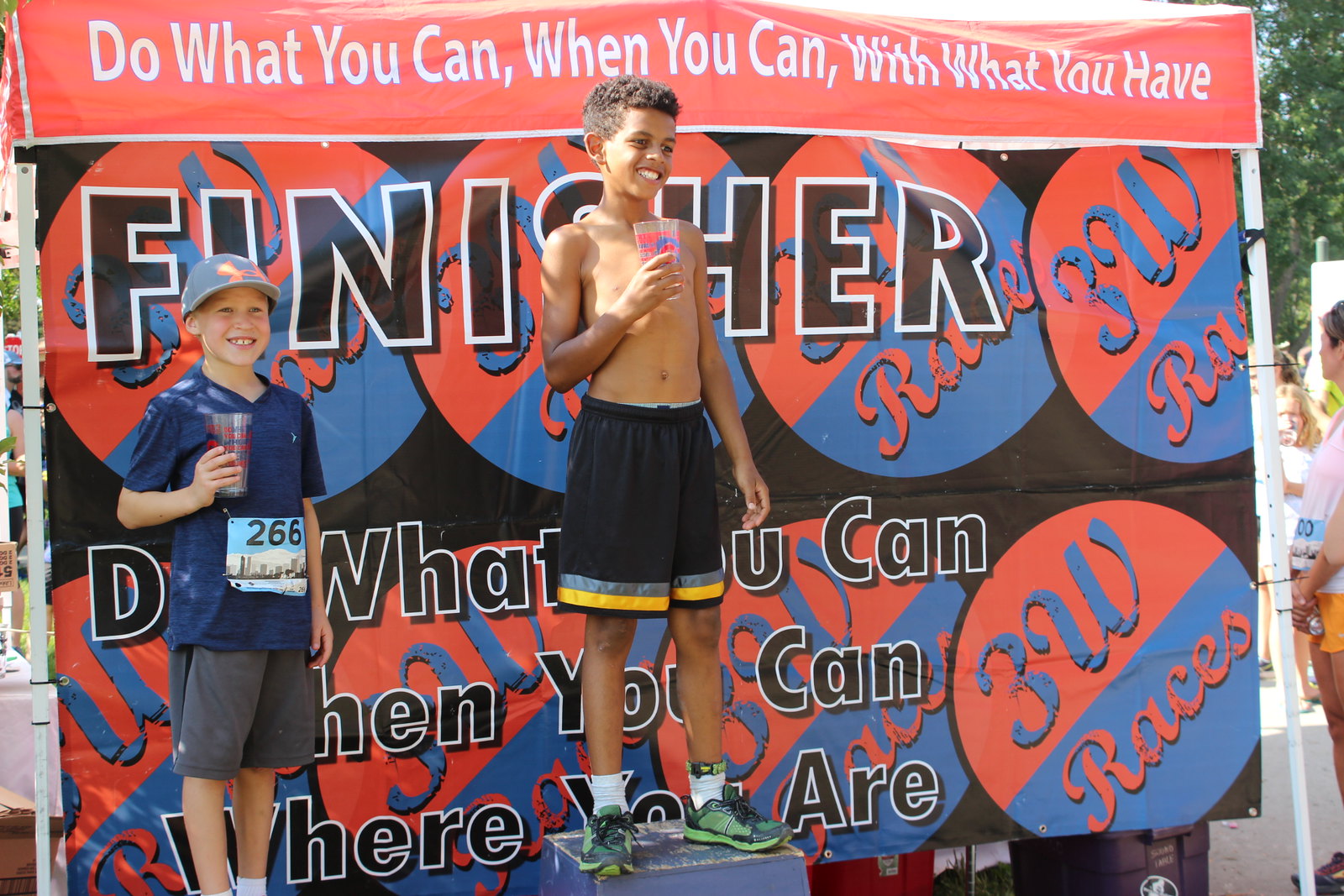In this vibrant outdoor scene, two boys, likely around 10 to 12 years old, stand proudly on a dark blue podium, celebrating their achievements in a race organized by 3W Races. The podium is divided into levels denoting their placements, with the taller level suggesting first place. Both boys are holding colorful plastic cups in their right hands, presumably their race trophies, and are beaming with joy. 

Behind them, an eye-catching banner displays motivational phrases in white lettering: "Do what you can, when you can, with what you have," and the word "Finisher" in bold black letters outlined in white. The banner also features the 3W Races logo, with the top half in red and the bottom half in blue, adorned with the word "races" in red cursive script.

The boy standing on the highest podium level has short brown hair and is shirtless, showcasing his athletic build. He is dressed in black shorts adorned with gray and yellow stripes near the knees and is sporting green running shoes paired with white socks. He is smiling broadly, clearly thrilled by his accomplishment. 

Beside him, at a slightly lower level, stands another boy with a number "266" pinned to his blue shirt, indicating his race number. He wears a blue hat with an orange Under Armour logo, gray shorts, and white socks. His plastic cup shares the same colorful design as his companion's, suggesting their shared victory moment.

The overall scene captures the exuberance and spirit of young athletes celebrating their hard-earned success.